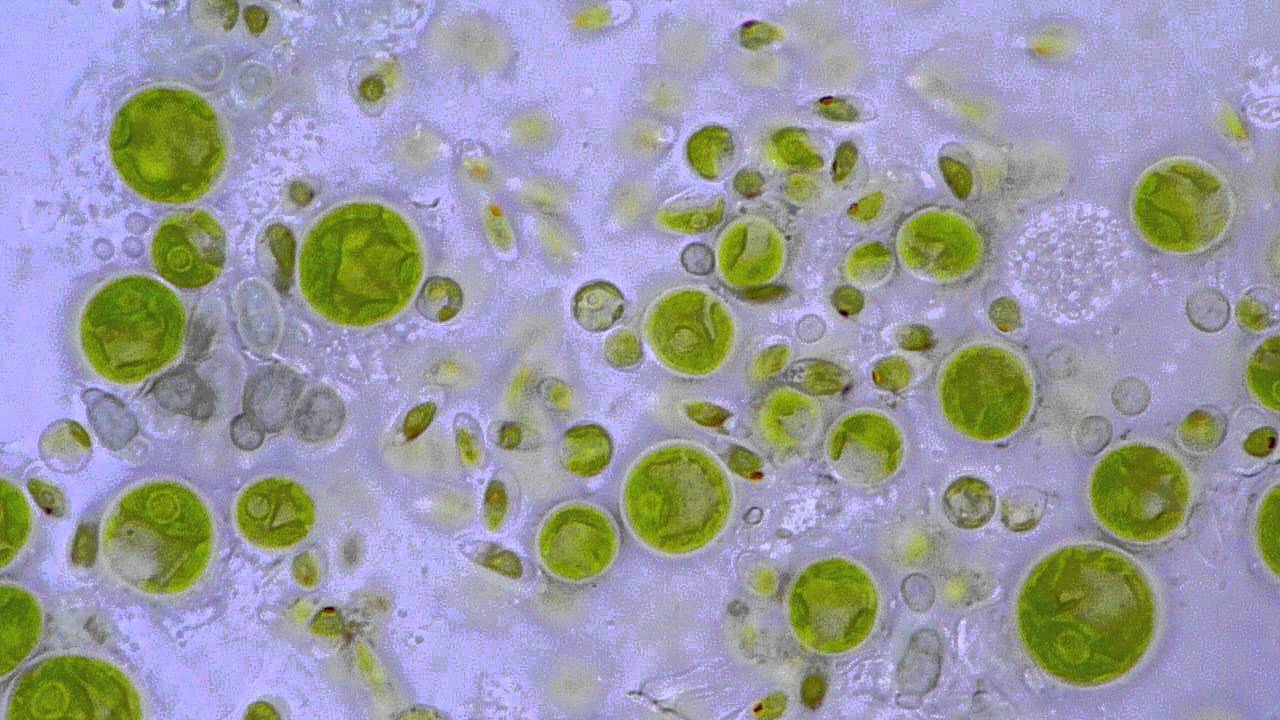The image is a magnified photograph taken under a microscope, showcasing a vibrant and intricate scene of green algae against a light purple, textured background. The predominant structures are round, green cells, some of which contain smaller particles within them, contributing to the detailed complexity of the image. The background exhibits darker purple shading on the edges, transitioning to a brownish, seed-like structure towards the center. Additionally, the purple background features diffused textures and circular, white patterns. A few of the green cells appear oval-shaped and slightly blurry, indicating they might be out of focus. The setting of the image is bright and clear, emphasizing the microscopic details despite some noise and pixelation due to the high magnification.